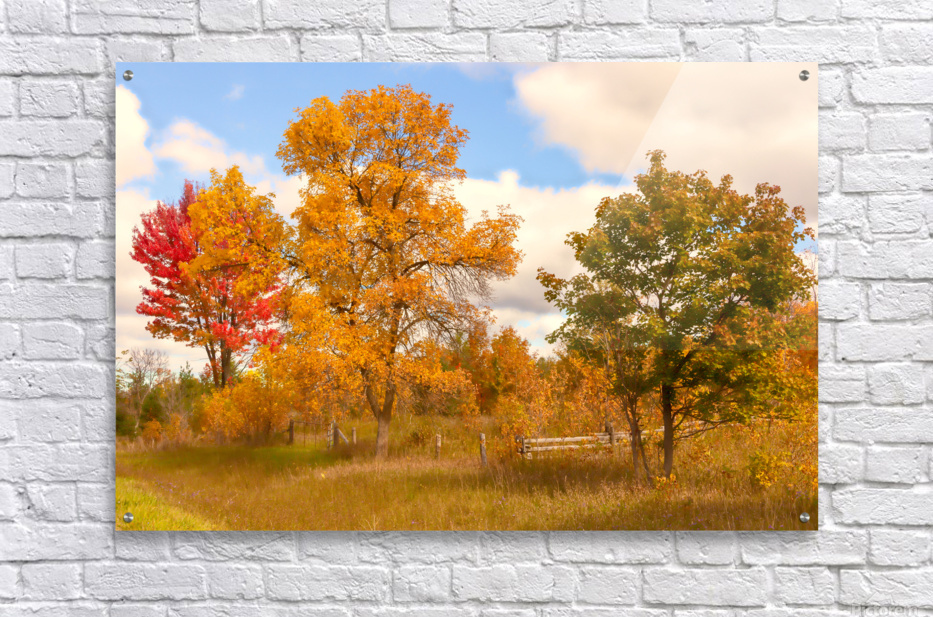The painting is mounted on a white-painted brick wall using four silver brad-type screws, one in each corner. Depicting a serene autumn day in a field, the scene features a wooden fence with brown posts and wire spanning between them. The grassy terrain is a yellowish-green, dotted with tall stems, indicating the transition of the season. Dominating the foreground are three vibrant trees along the fence line: the first tree displays green leaves tinged with yellow, the second is adorned with bright yellow foliage, and the third boasts vivid red leaves. Additional trees in the background exhibit a similar array of autumn colors. Above, the sky is a clear blue scattered with white clouds, encapsulating the crisp, peaceful essence of fall.